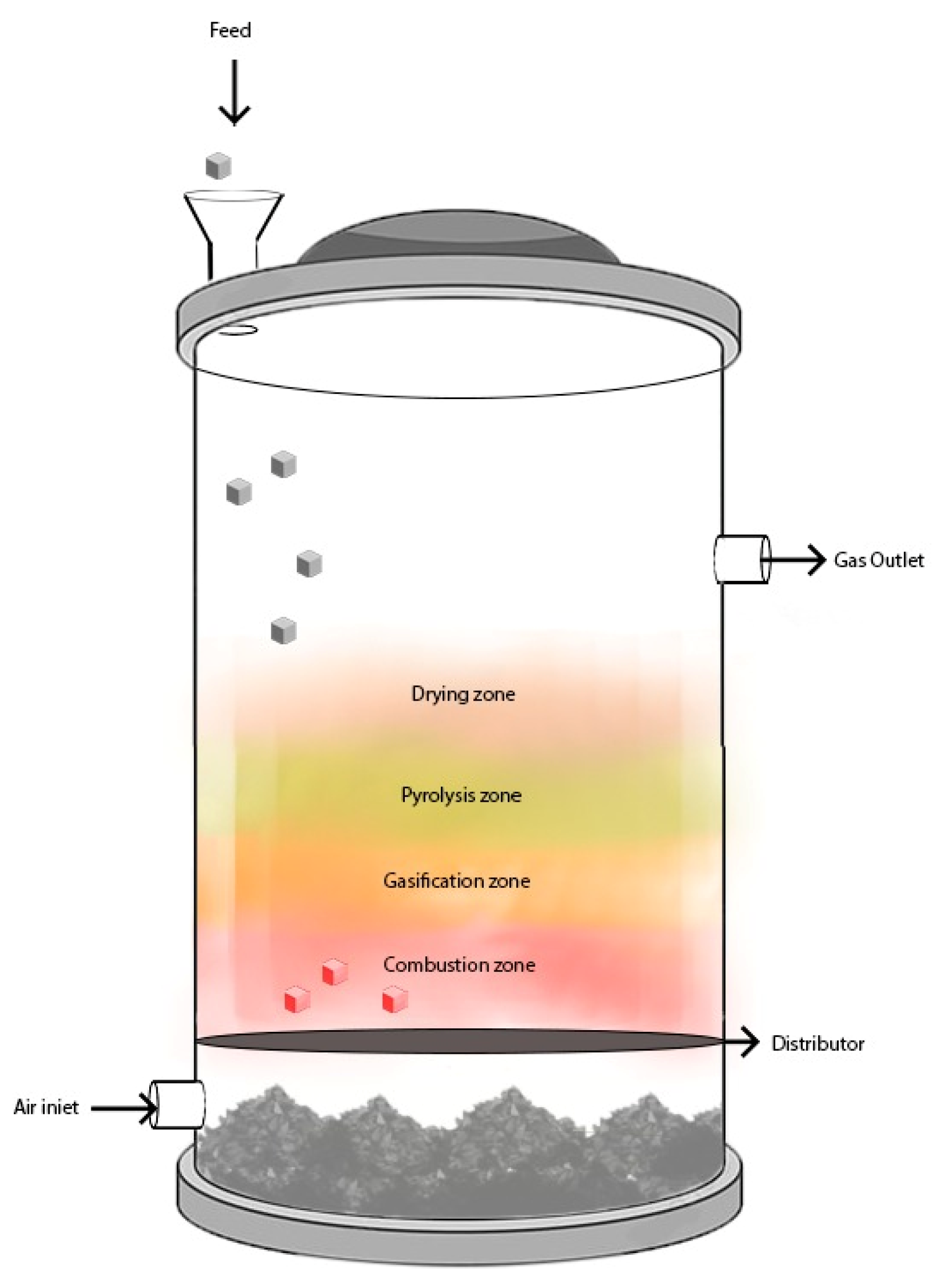The 2D illustration displays a detailed schematic of a process occurring within a cylindrical container on a white background. The container is divided into four distinct colored sections, each labeled to depict different zones: at the bottom is the reddish "Combustion Zone," above it is the "Gasification Zone" in orange, followed by the "Pyrolysis Zone" in green, and at the top is the peach-colored "Drying Zone." 

At the top of the cylinder, there is a labeled "Feed" inlet where small gray cubes labeled as feed fall in, guided by a downward-pointing arrow. The illustration also shows these cubes moving into the container. 

On the right side of the cylinder, there is a "Gas Outlet" with an arrow indicating the direction of gas flow out of the cylinder. At the very bottom of the cylinder, there is an "Air Inlet," where air presumably enters the system. The combination of these detailed components effectively displays the sequence and interaction of the different zones and the materials within this cylindrical system.